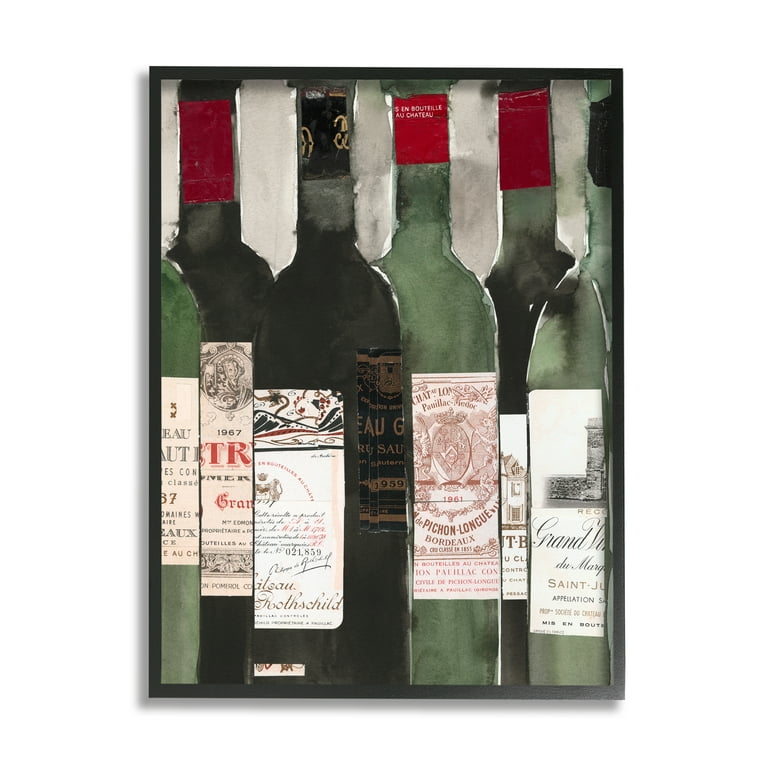The image is a detailed watercolor painting depicting six distinct wine bottles set against a tan-gray background. Four of the bottles are prominently visible, while the other two are partially cropped on the edges. The bottles feature various labels ranging in color from beige, tan, white, and peach, to cream. Their tops are adorned with colorful foil wrappers—one with a red wrapper, a top black, and two more reds. The bottles themselves are a mix of three green glass and three darker bottles that appear nearly black. The artwork is abstract, with labels positioned to mimic the form of bottles, and they bear partial, barely discernible text such as "Grand," "Deux," "Saint," "Paliac," "Medoc," "Pichon Long," and "Bordeaux," suggesting a variety of red wines. The painting's style is slightly crude and abstract, with a light shading around each bottle to imply reflections and edges.